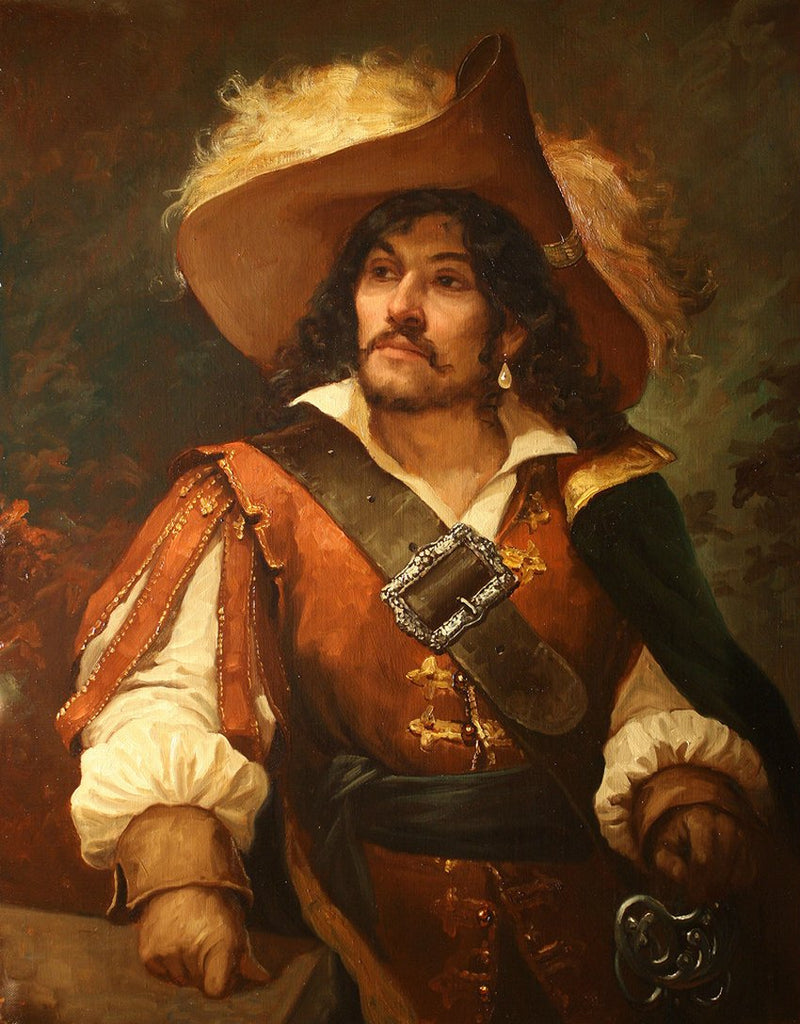This painting depicts a distinguished gentleman from the 16th or 17th century, adorned in period clothing that is rich with detail. He wears a wide-brimmed, floppy hat topped with puffy white fur, framing his long, curly black hair and a long, brown mustache. A white pearl earring dangles from his ear. His penetrating gaze is directed off to the left side of the frame. He sports an off-white poet's shirt with voluminous sleeves, coupled with light brown gloves, and a red vest that extends downward. Draped across his right shoulder, descending to his left waist, is a thick leather belt featuring a large silver buckle. Over his left shoulder, a luxurious green and gold cloak adds an air of opulence. Completing his attire, a dark green ribbon cinches his waist. His right hand rests upon a wooden structure, while his left hand grips the hilt of a sword, grounding him in a commanding pose. The background consists of abstract splotches of green and red, complementing the vibrant colors of his clothing.